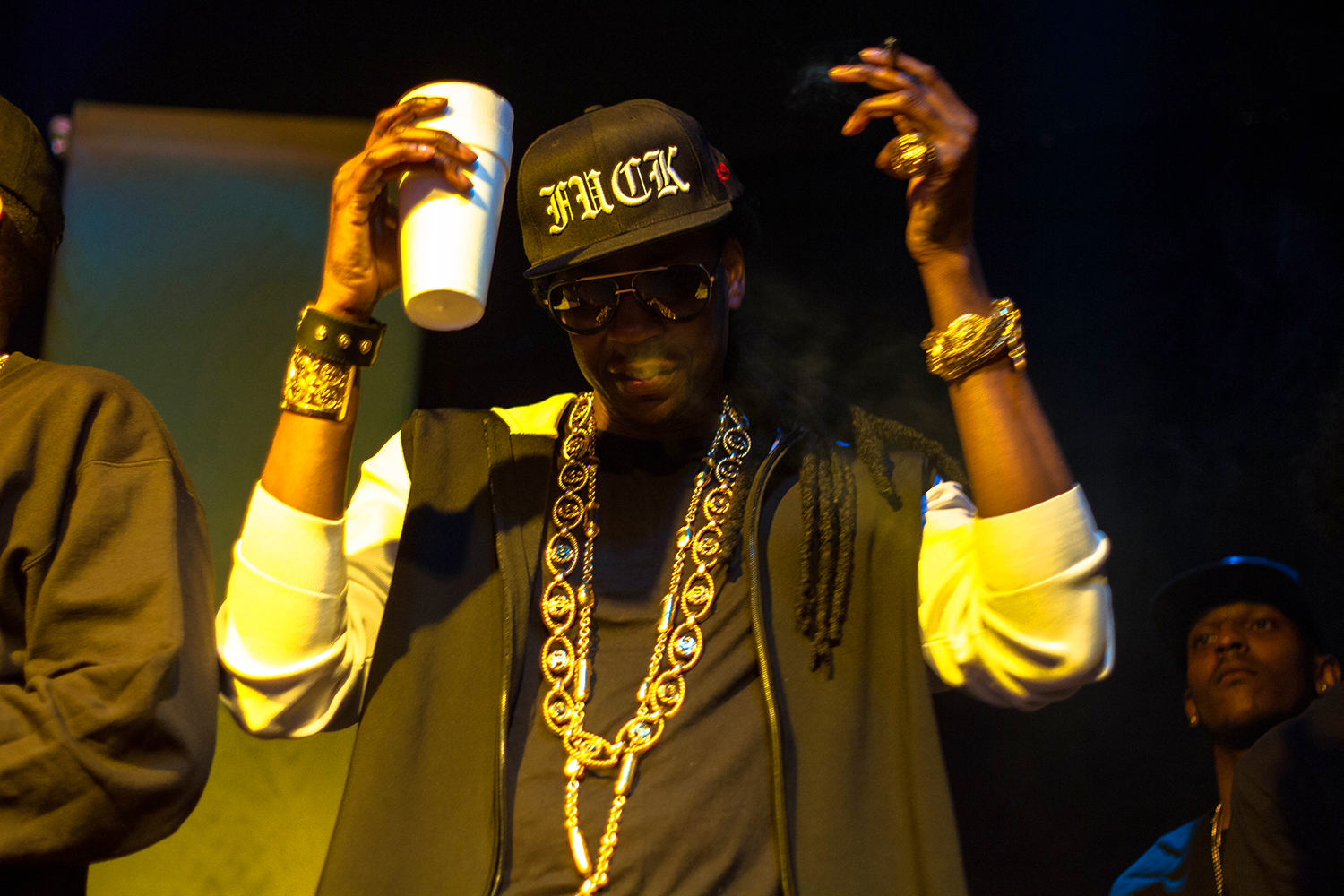This photograph captures a young Black male, possibly a rapper, enjoying himself at a social event, either a concert or a sporting occasion. Positioned at the center of the image, he is shown from mid-waist to the top of his head. He wears a black baseball cap with the word "F-U-C-K" emblazoned in Old English style lettering. His attire includes a brown vest over a white long-sleeved sweatshirt, with a brown shirt peeking from underneath. Heavy gold chains drape around his neck, and he's adorned with multiple bracelets—gold on both wrists, and an additional black leather bracelet or watch band on his right wrist. 

Aviator sunglasses obscure part of his face, but his expression suggests he's either smiling or engaging in lively conversation or song. His arms are bent at the elbows, with his forearms raised upwards. His left hand appears to be making a snapping gesture, while his right hand holds a white styrofoam cup high, just above the level of his head. 

His overall look is completed with long, braided dreadlocks. The backdrop suggests an indoor setting with a blue wall and yellow lighting on the left side. The shoulder of someone wearing a black sweatshirt appears on the left side of the image, while another Black male, donned in a baseball cap and blue jacket with a gold necklace, is distantly visible at the lower right corner. Smoke trails from his mouth, indicating he might be smoking a blunt in his left hand. The combination of his stylish attire and the ambient lighting lends an energetic and vibrant atmosphere to the photograph.